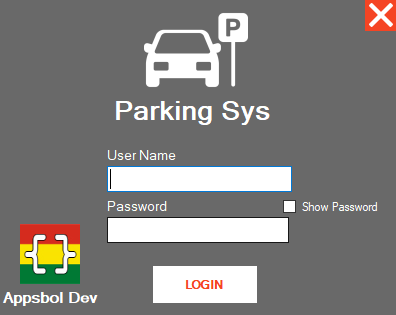The image depicts a user interface for a parking system. Prominently featured in the top-right corner is a red box. Below this, the interface includes a username section characterized by a large input bar, delineated by a vertical black line indicating where the user can enter their username. Adjacent to this section is a password input field marked with the text "Password." A checkbox labeled "Show password" is situated nearby, allowing users to toggle the visibility of their password.

At the bottom left corner of the interface, the text "Apps Full Dev" is displayed. Just above this text, there is a colorful square divided into red, yellow, and green sections, enclosed within square brackets.

The log-in button is a white rectangle with bold red text reading "Log In." In the upper portion of the interface, icons for a car and a parking sign underscore the purpose of the system—managing parking.

Overall, this layout presents a simple yet functional log-in system for users aiming to access a parking management application.